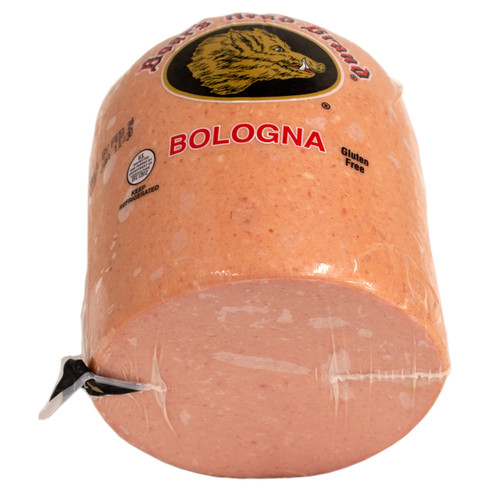The image depicts a cylindrical, thick chunk of Boar's Head brand bologna, clearly encased in shrink-wrapped plastic. The background is a stark white, drawing attention to the bologna itself. The front-facing slice of the bologna reveals its reddish-orange flecked color. The packaging is seamless, with visible plastic seams at the bottom. Prominently displayed at the top of the package is the Boar's Head logo, featuring an animated brown boar on a black circular background. The logo is surmounted by the Boar's Head Brand name in Old English red and black font. Below the boar's head, "bologna" is inscribed in bold red letters with a white outline. To the right of "bologna," the packaging indicates "gluten-free" in small black font. To the left, there's a USDA inspection symbol and an expiration date, which is somewhat obscured. The logo, branding, and essential information all encircle the cylindrical shape of the bologna, making the packaging both informative and visually distinctive.